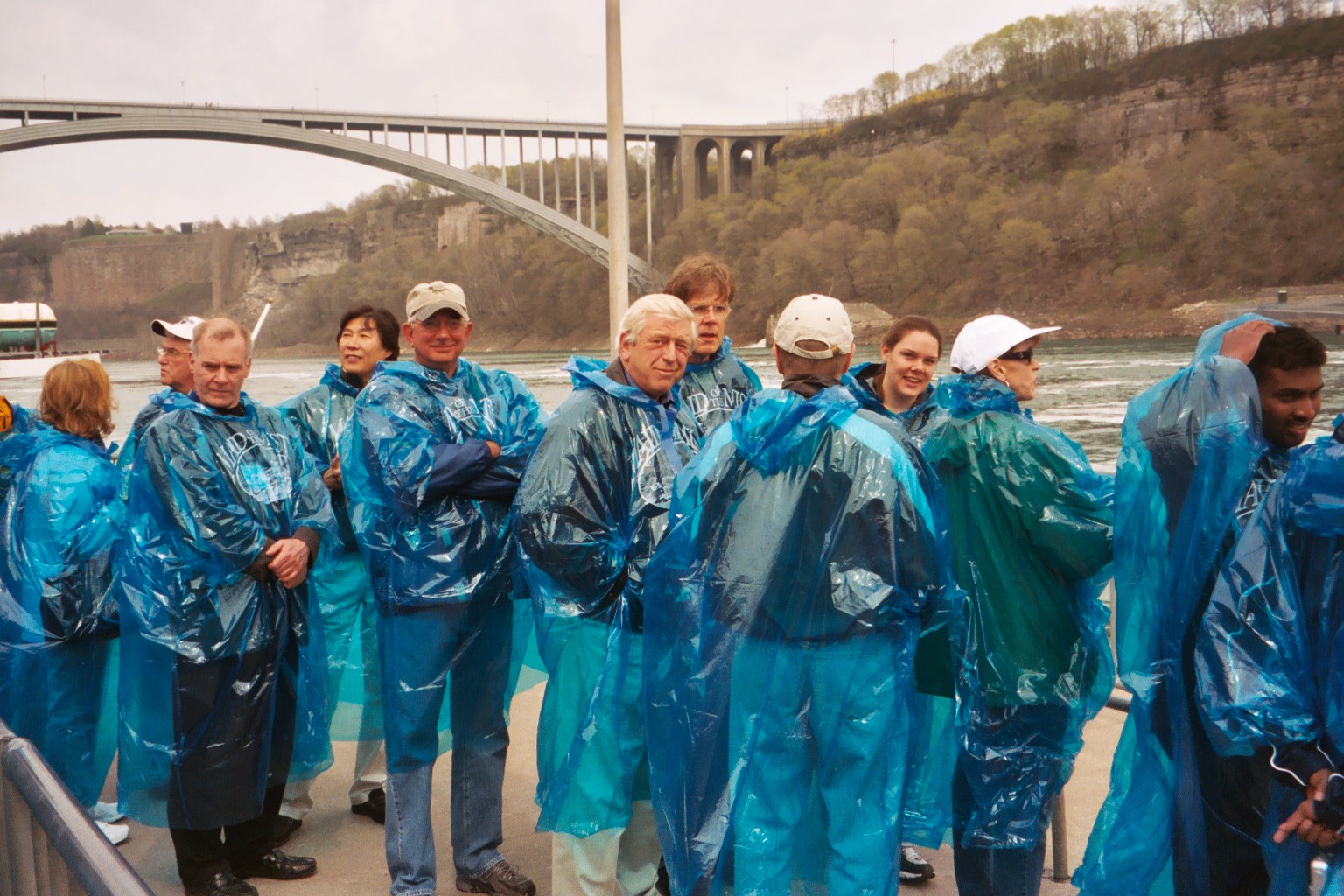The photograph captures a diverse group of mostly older adults, comprised of men and women of various races, standing at the edge of a river beneath an overcast sky. They are outfitted in inexpensive, hooded blue ponchos, making them appear as though they are ready for an excursion, possibly in a spray-heavy area like Niagara Falls. In the background, there is a prominent, large, silver-gray steel bridge with an arch, spanning over the water. Beyond the bridge, the other side of the river features a high, rocky bank topped with a tree line. The landscape includes a big brown mountain adorned with trees. Among the crowd, a man with jeans and crossed arms stands out, looking directly at the camera, alongside two other individuals also making eye contact with the lens. The group seems to be waiting in line, and the photograph has a mild sepia tone that imparts a slightly dated feel.